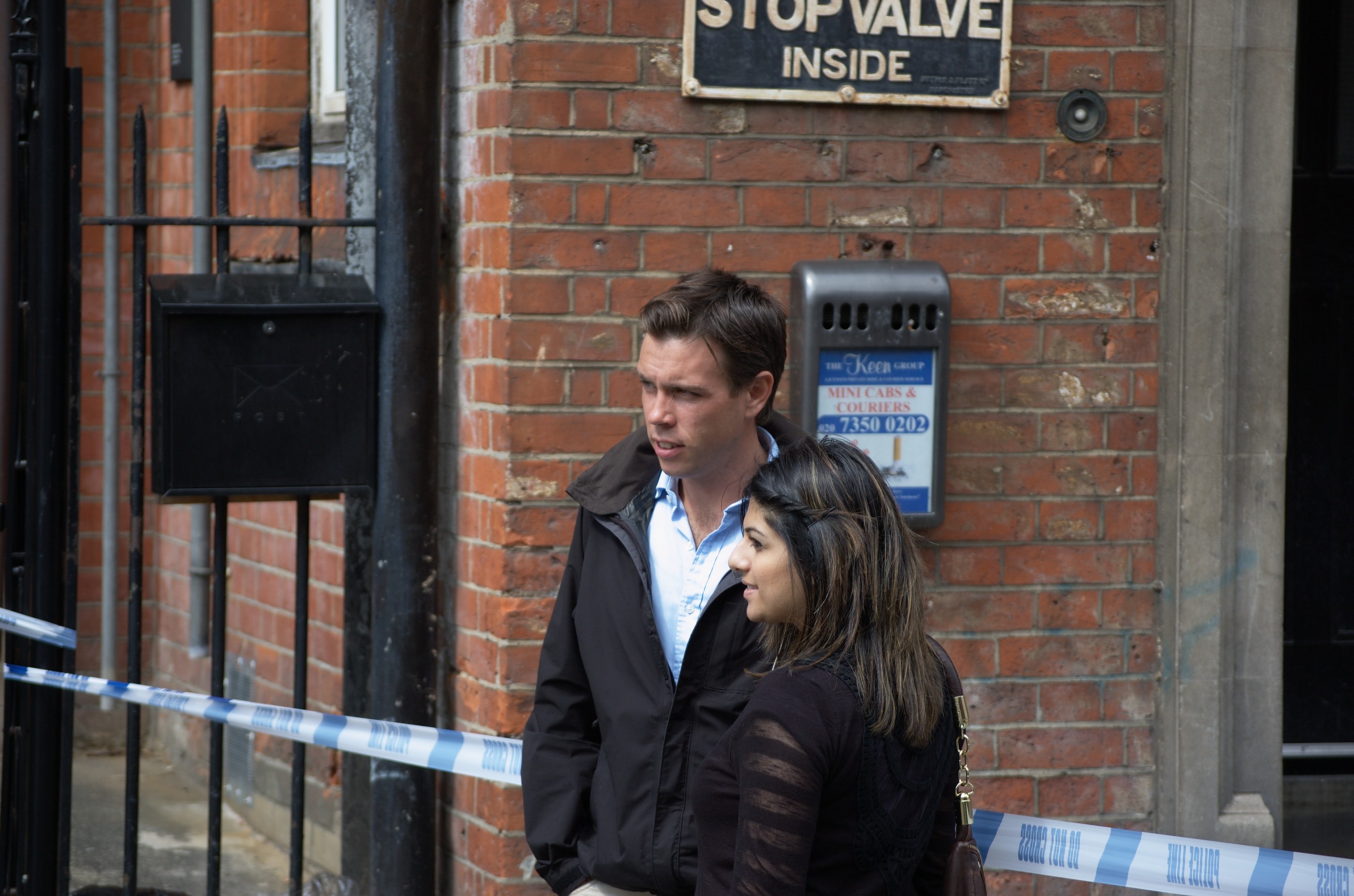In this photograph, there are two young adults, likely in their early 20s, standing in front of a weathered red brick building in an urban setting. The man, with short brown hair, is wearing a light blue shirt and a black winter jacket zipped up. The woman, sporting long dark hair, is dressed in a black top and carries a brown purse. Both of them are looking off to the left in the distance. A blue and white striped "do not cross" tape is affixed nearby, suggesting an area restriction. Behind them, a black rectangular sign with gold lettering and accents reads "stop valve inside." A brown metal box is attached to the building, possibly a mailbox or an advertising sign, while another black box, likely another mailbox, is mounted on a metal bar fence.